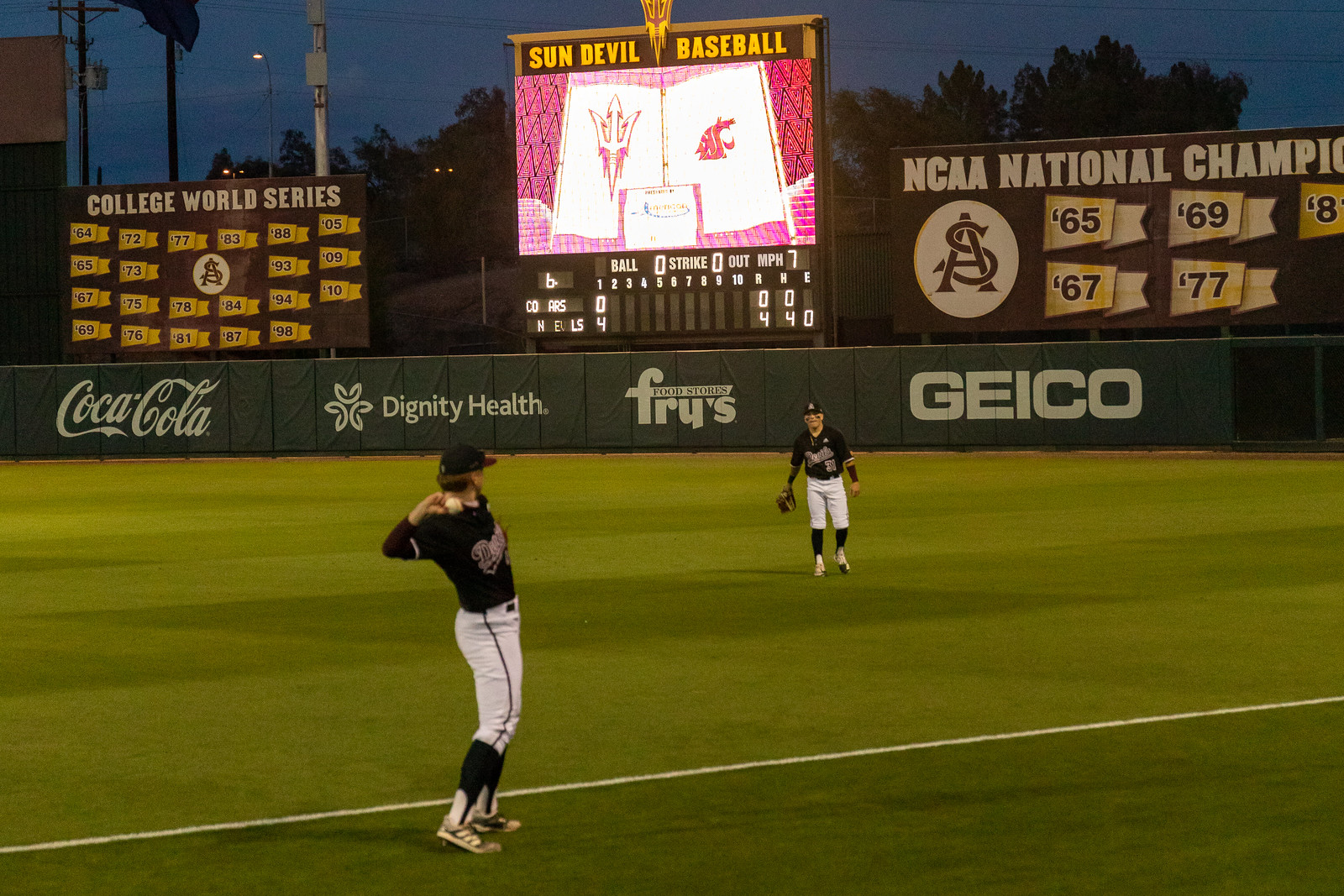This horizontally aligned rectangular picture captures an Arizona State Sun Devil baseball game at Sun Devil Stadium. Two players are engaged in warm-up tosses, one positioned in foul territory while the other stands in the outfield, both wearing the team's uniform of white pants with a black stripe and a black jersey. The player in the foreground, turned away from the camera, is poised to throw the ball held in his right hand. They are standing on green turf marked by a white line. 

In the background, prominently displayed on the outfield wall, are white logos for Coca-Cola, Dignity Health, Fries, and GEICO. Above these ads, several signs highlight the stadium’s historic achievements. There's a banner for the College World Series adorned with yellow flags and corresponding numbers. To the right, another banner celebrates NCAA National Championships with years '65, '67, '69, '77 listed against yellow flags, featuring a circular white logo with an "A" and an "S" layered on top. Central among these signs is the scoreboard, indicating the game between the Arizona State Sun Devils and the Washington State Cougars, with the score showing a 4-0 lead for the Sun Devils after one inning.